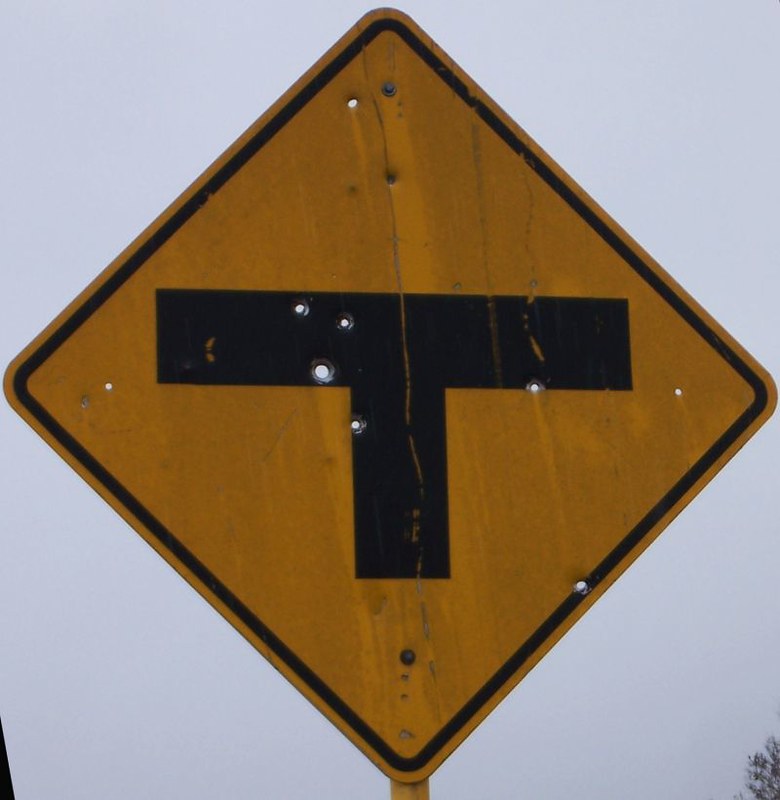Captured in this photograph is a weathered and old diamond-shaped street sign, boasting a mustard yellow background. Central to the sign is a thick, black "T" with an elongated top, a hallmark of a road intersection warning. Scattered across the sign are numerous bullet holes of varying sizes, giving it a rough and battered appearance. Cracks in the paint and streaks of dirt further enhance the sign's aged and worn look. The sign is outlined with a thin black border and is mounted on a partially visible yellow pole. In the lower-right corner of the image, the silhouette of a tree's tip just barely intrudes, against a backdrop resembling a cloudy sky, adding a touch of nature to the scene.